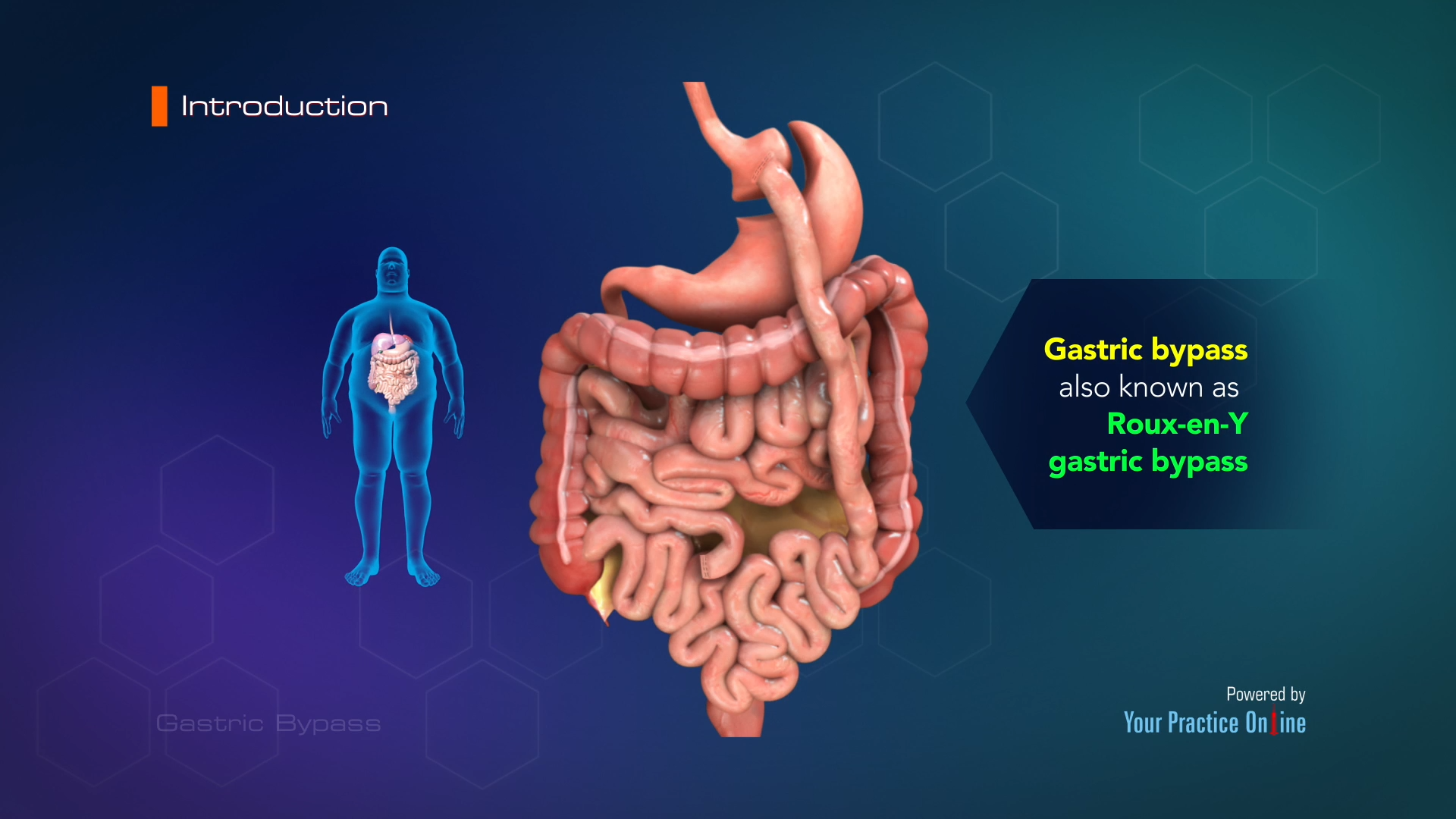The image appears to be an introductory slide from an online lecture or presentation about gastric bypass surgery. At the top left corner, a red-orange bar labels the section as "Introduction." Beneath this, two images are displayed. The image on the left features a blue silhouette of an obese person, with an X-ray-like view of their digestive system, including the esophagus, stomach, and both large and small intestines. This visual representation is somewhat cartoonish yet detailed. On the right side, there is a close-up view of the digestive tract, showcasing an animated and realistic depiction of the stomach and intestines in a pinkish-beige color. Both images relate to the topic of gastric bypass, which is emphasized by the text "Gastric Bypass" and "Also known as Roux-en-Y Gastric Bypass" in yellow and green, respectively. The bottom right corner features a faint caption that credits "Powered by Your Practice Online."